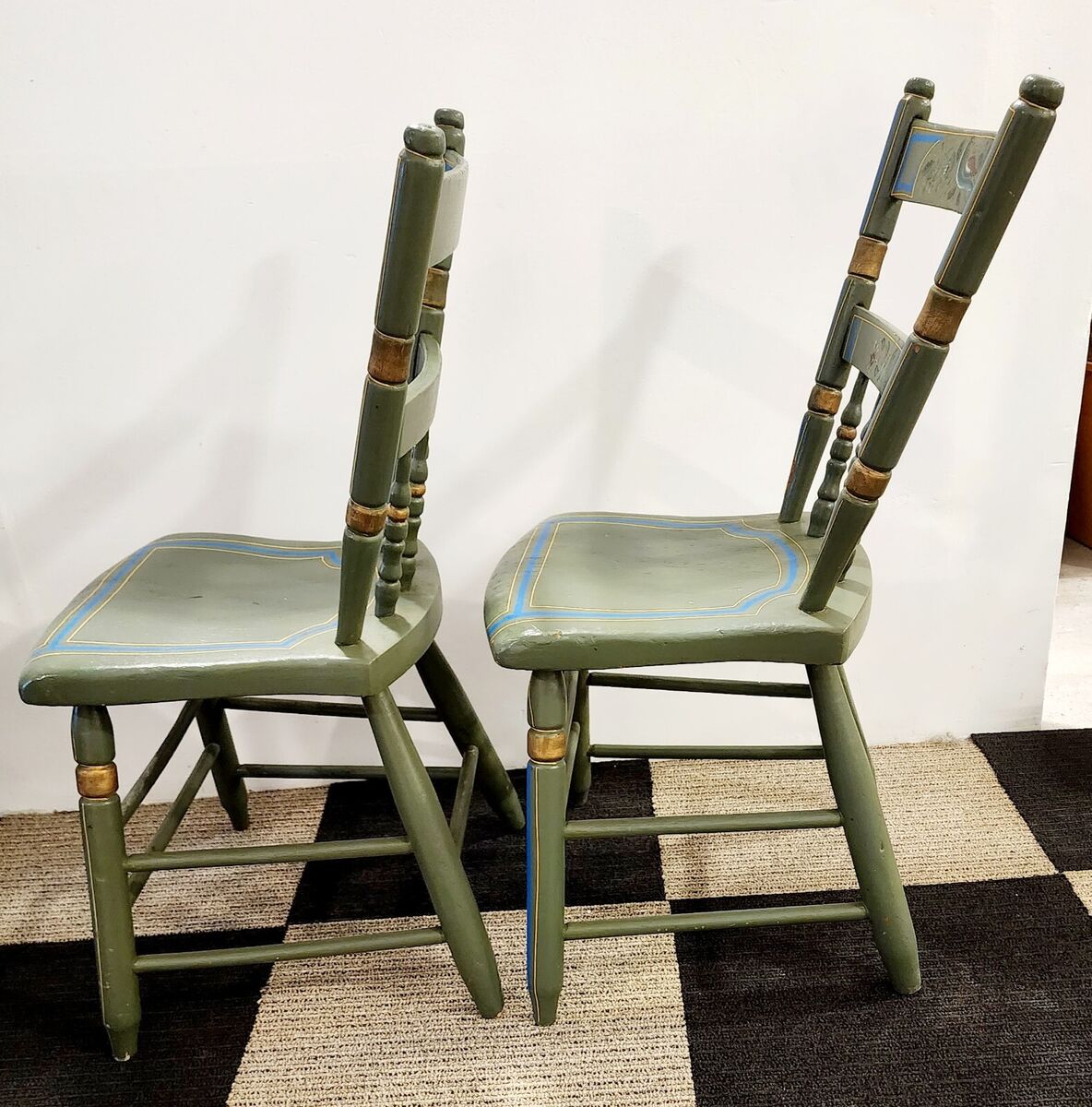In the photograph, we can see two chairs positioned against a white wall, one chair slightly in front of the other. The chairs are predominantly olive green with brown accents, featuring golden hues on the legs and backrest. The seats of the chairs are outlined with blue and yellow, and the backrest is adorned with a colorful design incorporating blue, green, and red elements. These wooden chairs, with no armrests, have four legs each. They are placed on a checkered rug with a black and yellow pattern. A small part of another room is visible in the bottom right corner of the image.